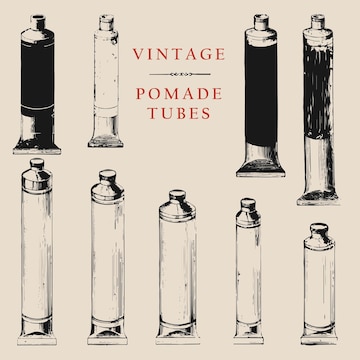The poster features a vintage design reminiscent of the early 20th century, with a light pink or beige background. At the center, in bold red letters, it reads "VINTAGE POMADE TUBES," printed in an all-capitalized font similar to Times New Roman. Surrounding this central text, there are nine illustrations of pomade tubes arranged symmetrically. At the top, two tubes on each side of the title are placed vertically, with some tubes being predominantly black and others being mainly white, all with contrasting details. These tubes resemble those used for oil or watercolor paint, complete with caps at the top. At the bottom of the poster, five additional tubes are displayed, varying in length from the tallest on the left to the shortest on the right, also in similar black and white styles. The tubes at the bottom have black tops and bottoms. Overall, the poster is square-shaped, evoking a classic, vintage aesthetic that highlights the varied designs and lengths of the pomade tubes.